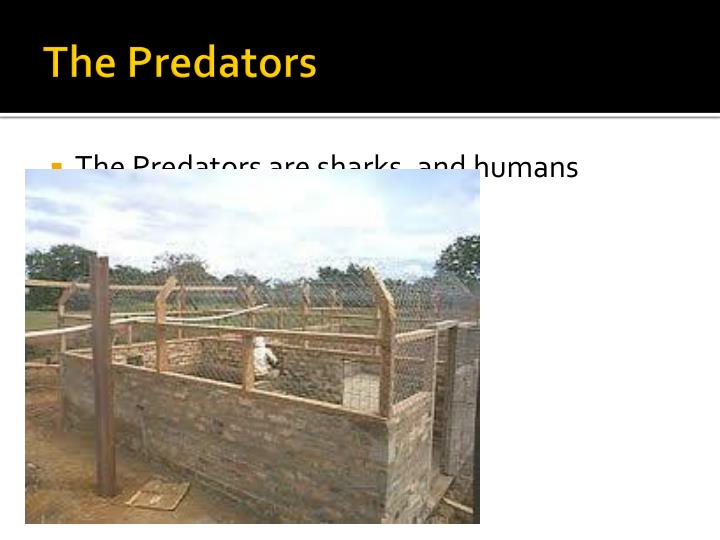The image consists of a top section featuring a solid black band that spans from left to right. Centered within the black band is the phrase "The Predators" in gold text. Just below this band runs a dark gray line across its entire length. Underneath, there is black text on a white background that reads, "The Predators are sharks and humans," preceded by a small yellow bullet point. Slightly obscuring this text is a prominent square photograph, creating the impression of being somewhat out of place. The photo depicts an outdoor enclosure with a dirt floor, encircled by a brick wall topped with a chain-link fence. In the background, beyond the enclosure, are green trees and a blue sky. Within this confined space stands a figure, possibly a man wearing a white shirt, seemingly confined within the makeshift cage-like structure.